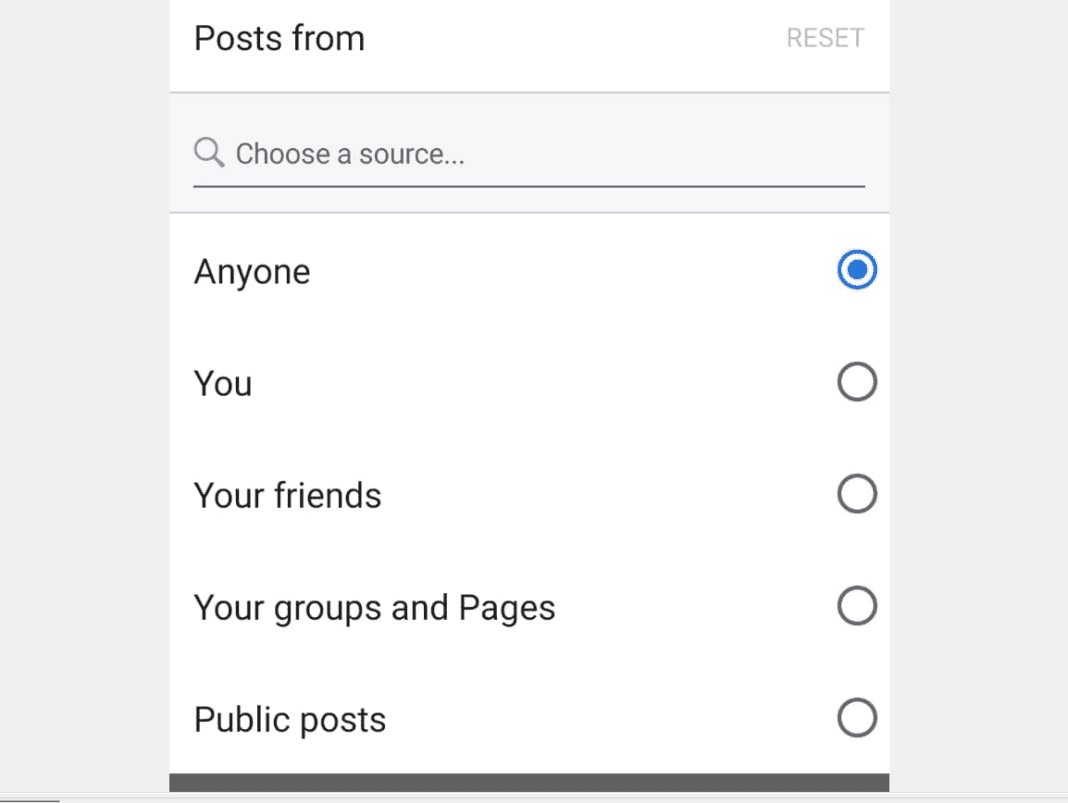The image features a user interface template set against a white background, framed by a darker gray outer border. At the top of the image, a heading reads "Posts From," flanked on the right by a "Reset" option in thin, gray text. Directly beneath this heading is a long rectangular search bar labeled "Choose a Source," accompanied by a magnifying glass icon on its left. A horizontal line separates this search area from the filtering options below.

The first filter category below this line is labeled "Anyone," with a blue circle to its right, indicating it is currently selected. Successively, there are additional categories titled "You," "Your Friends," "Your Groups and Pages," and "Public Posts." Each of these has a corresponding open circle to the right, signifying that these options are not selected. 

At the very base of the image, another horizontal line spans the width of the page in dark gray. This entire layout is superimposed on a light gray background, providing a subtle contrast to the primary white backdrop of the interface elements.